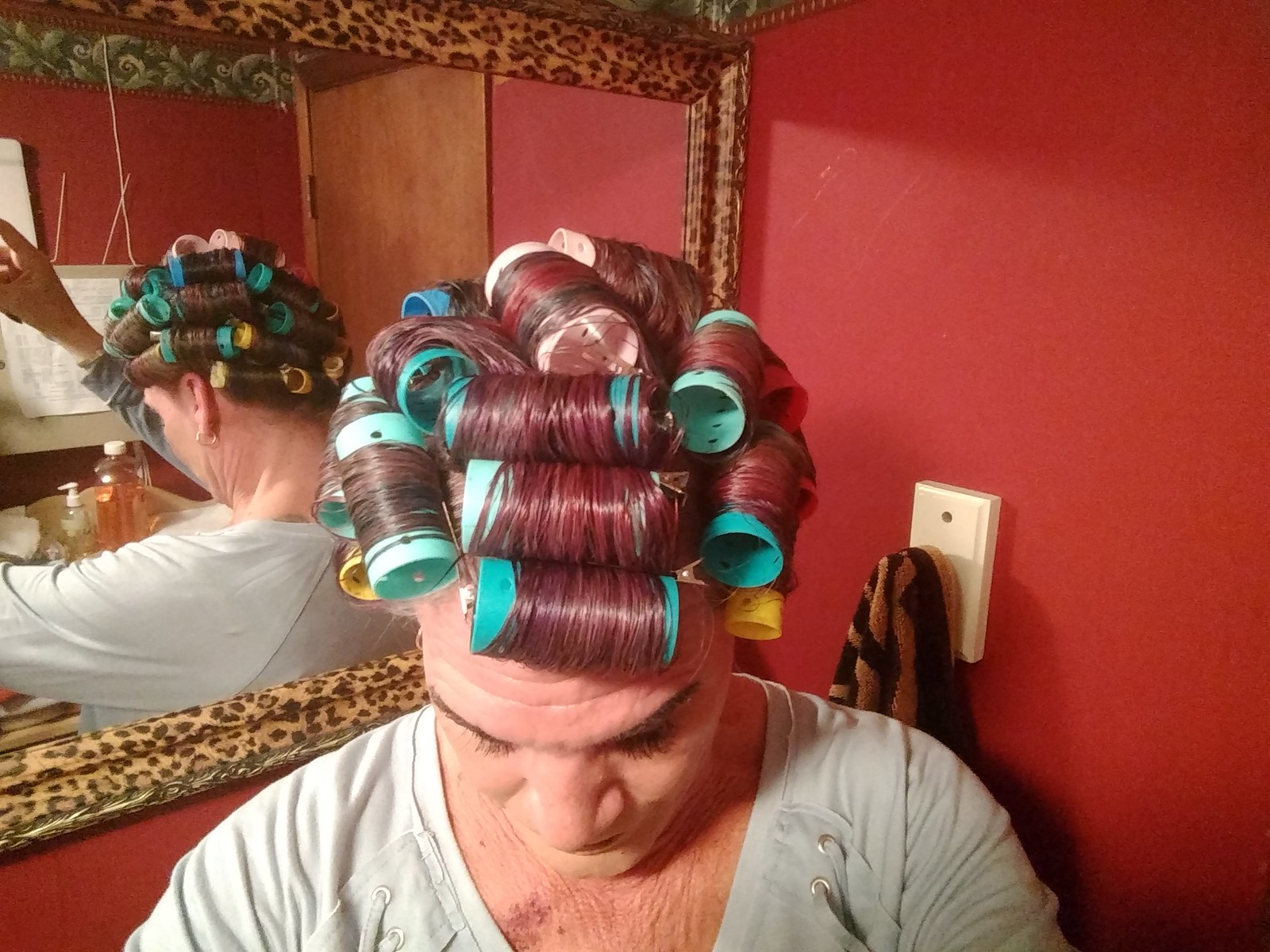The image depicts a close-up photograph of an older woman with dyed auburn burgundy hair, styled in numerous curling rods. Most of the curlers are teal, with some white and two yellow ones. She is taking a selfie, leaning her head forward to capture the top of her head. Her hand holding the camera is not visible. The room's walls are red, and there is a mirror behind her with a cheetah-print border frame. In the mirror's reflection, you can see the back of her head and her arms raised to take the picture.